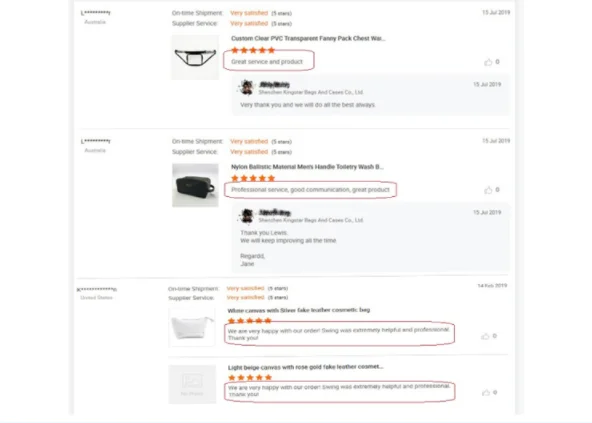The image appears to be a blurred screenshot or graphic with a white background and a gray horizontal border running across it. The text, which is difficult to read due to the blurriness, seems to detail various products alongside customer reviews and ratings. Key information includes:

1. **Clear PVC Transparent Fanny Pack**:
   - Review Date: Either June or July of 2001, or possibly 2018 or 2019.
   - Rating: Five stars.
   - Review: Enclosed in a red border, stating "Great service and product."

2. **Nylon Handle Toiletry Wash Bag**:
   - Review Date: Likely the same as the fanny pack review.
   - Review: Enclosed in a red border, stating "Professional service, good communication, great product."

3. **White Cosmetic Bag**:
   - Description: Contains the word "white" and seems related to cosmetics, though specifics are unclear.
   - Review: Enclosed in a red border, stating "We are very happy with our order," followed by "extremely helpful and professional, thank you."

At the top, there are sections labeled with the words "on-time shipment" and "supplier service" in black, and a note of "very satisfied" in orange. The overall theme indicates positive feedback on service and product quality.